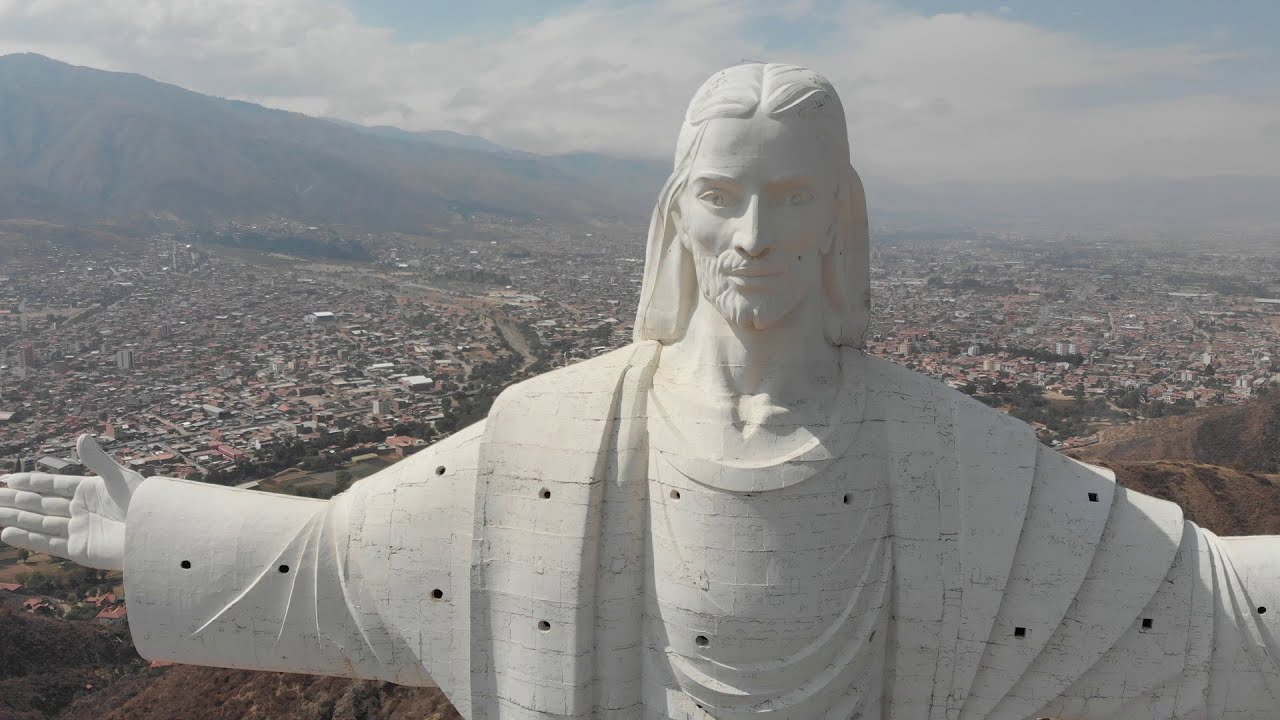The image prominently features an up-close view of the iconic Christ the Redeemer statue in Brazil. The statue, sculpted from white stone and depicting a male biblical figure with long hair, a beard, and outstretched arms, occupies the foreground. The framed view captures the statue from its right hand in the lower left corner up to the head in the image's center, extending only to the elbow of its left arm in the lower right corner. Set atop a hill, the statue overlooks a highly urban cityscape of predominantly white, tan, and gray buildings, stretching from residential areas with rolling houses to distant skyscrapers. A large road snakes through the middle of the city, partially visible over the statue’s shoulder. In the background, a mountain range rises beneath the cloudy blue sky, which is tinged with smog or haze, adding to the slightly obscured, misty atmosphere.